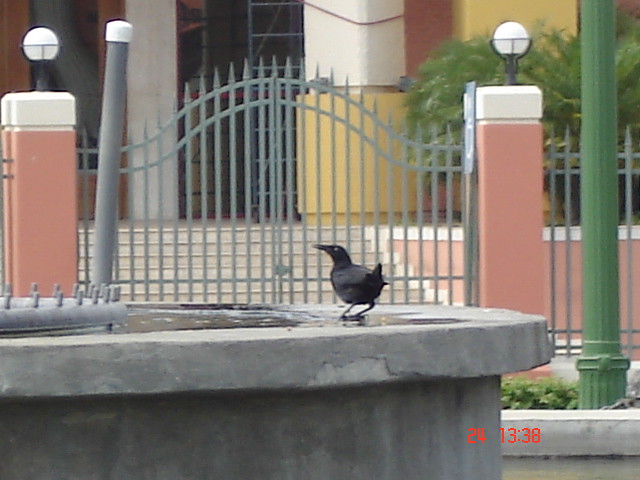The photo captures an outdoor scene featuring a black crow perched on the edge of a circular cement water fountain, which stands about three and a half feet high. This fountain, though currently not operating, reveals several spigots sticking up into the air. The bird, with its long, sharp beak, appears to be looking around cautiously. Surrounding the fountain, the area is detailed with several architectural components: concrete columns painted red and a yellow concrete building in the background. A wrought iron fence with a double gray arch gate leads to steps that ascend into the building. These columns support a round lamp on each side, crowned in white and red paint. A green metal lamppost and a blue handicap sign are also visible near one of the columns. Additionally, at the bottom of the picture, red numbers "24, 13, 38" are inscribed.